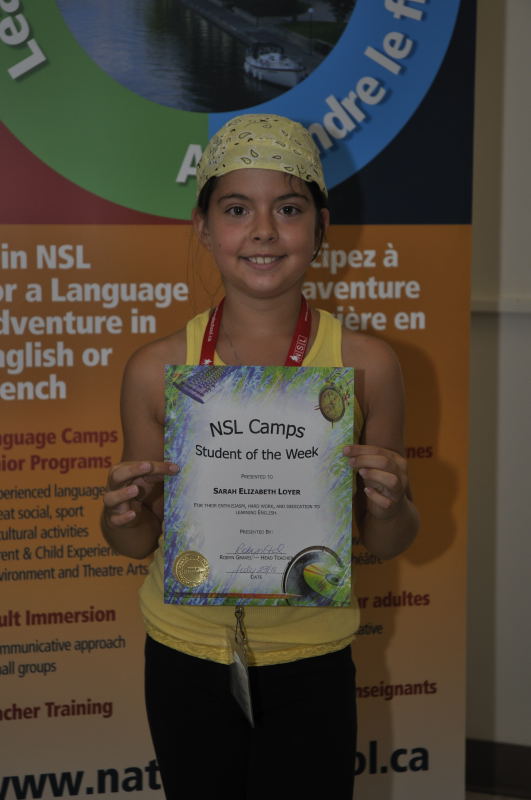In this indoor image, a young girl, around eight years old, stands beaming with pride as she holds up a certificate in front of a large, colorful poster. The poster, filled with hues of green, blue, and orange, prominently features white lettering with phrases such as "NSL," "Language Adventure," "Language Camps," and mentions of social, sport, and cultural activities, indicating it is from a language camp. The girl, with bright eyes and a dazzling smile, is adorned with a yellow bandana on her head, a yellow tank top, and a red lanyard around her neck over black pants. The certificate in her hands proudly reads "NSL Camp Student of the Week, presented to Sarah Elizabeth Lawyer," complete with additional text and a gold medallion in the lower left corner.